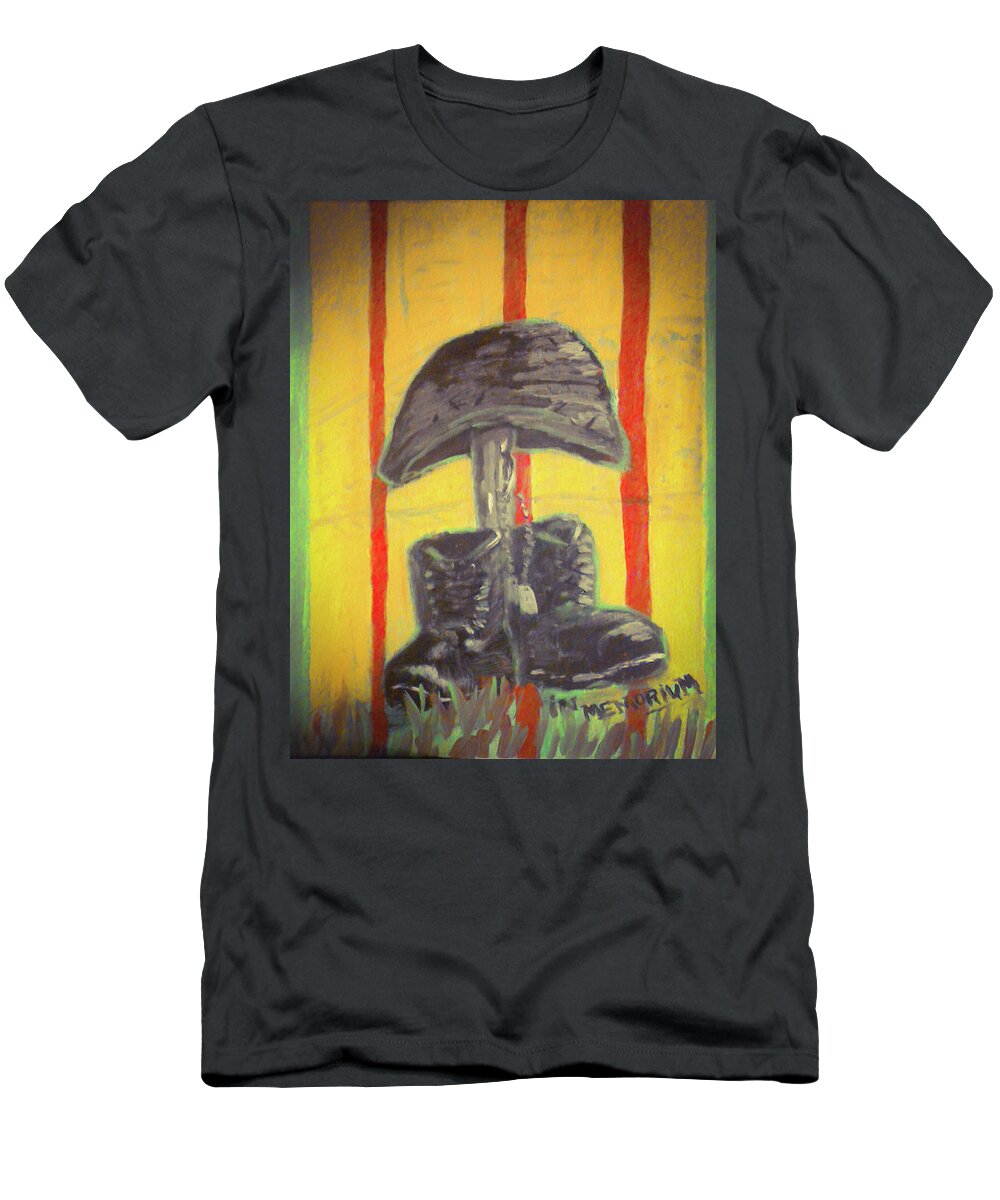This photo features a black t-shirt displayed on a white background. The centerpiece of the t-shirt is a rectangular print with alternating vertical stripes in green, yellow, and red; the yellow stripes are notably thicker compared to the green and red ones. Inside this rectangular section, a detailed painting-like image captures a somber tribute: a pair of black combat boots with laces are grounded at the base, and a stake or stick rises from them. An army helmet is placed atop the stake, while a dog tag hangs from a nail on the stake, suggesting the boots belong to a fallen soldier. The background of this scene subtly incorporates elements resembling grass, and the visuals are highlighted with white brushstrokes, adding a painted texture. At the bottom right corner of the rectangle, the words "In Memoriam" are inscribed, underscoring the t-shirt's intent as a tribute to those who have passed away, likely in military service.